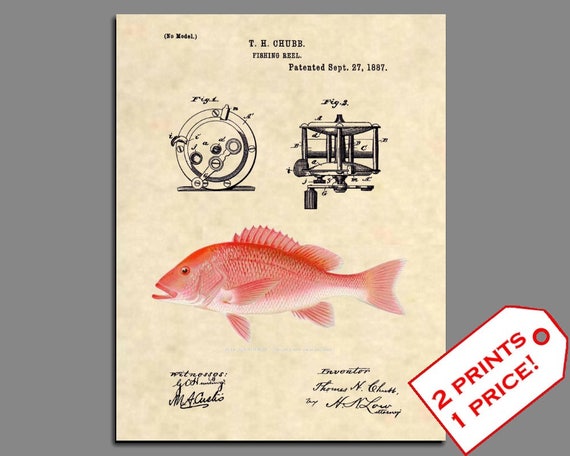The image is a detailed reproduction of an old, slightly worn beige piece of paper against a gray background. At the top left corner, the text reads "No Model" in black lettering. Centrally, it says, "T.H. Chubb Fishing Reel" and notes the patent date as "September 27, 1887." Below, there are architectural-style diagrams of the fishing reel, illustrating both side and top views. Beneath the diagrams, there's a depiction of a vividly colored, red-pink fish, likely a rock cod or bottom feeder, with its fins spread out. At the bottom of the paper, in cursive, are some hardly legible signatures. In the lower right corner, there's a white price tag with a red border that declares, "Two prints, one price." Overall, the image resembles a combination of a historical document and an artistic print.